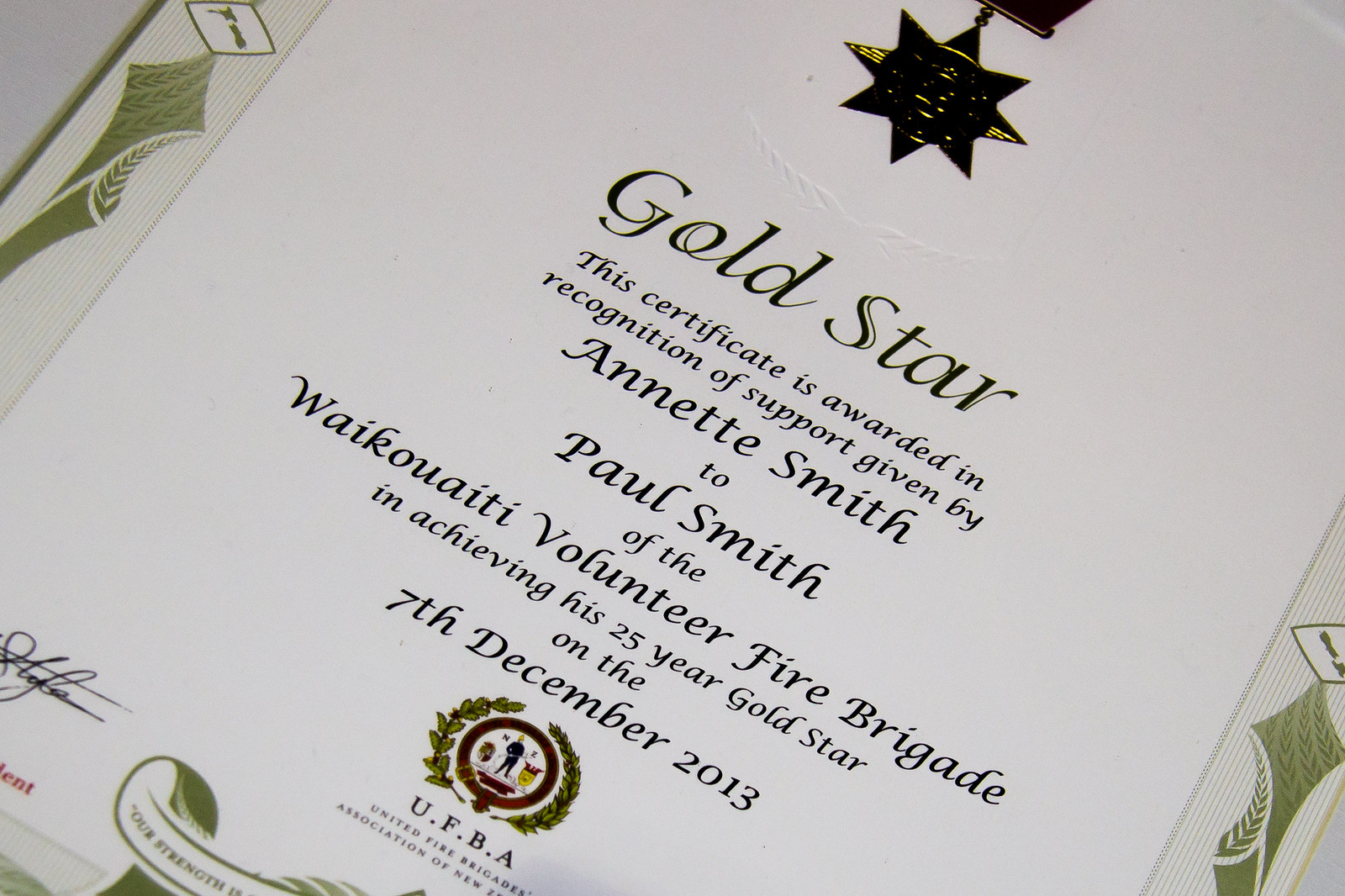The image captures a close-up, slightly tilted photo of an award certificate on white paper with gold-styled framing. At the top center, a gold star badge is prominently displayed. Beneath the badge in gold and black lettering, it reads "Gold Star". The text of the certificate, written in black cursive, states: "This certificate is awarded in recognition of support given by Annette Smith to Paul Smith of the Waikouaiti Volunteer Fire Brigade in achieving his 25-year Gold Star on December 7, 2013." Below the main text is an emblem accompanied by the initials "UFBA", likely standing for the United Fire Brigades Association of New Zealand. The bottom left of the certificate features a signature, and there's some additional, partially visible imagery at the lower center of the photo.